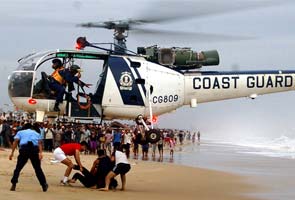The photograph captures a Coast Guard rescue operation on a beach with beige-colored sand under a gray sky. Central to the image is a white helicopter with blue trim, bearing the words "Coast Guard" and "CG-809" on its tail. The helicopter hovers just above the sand, indicating an active emergency. In the forefront, four individuals focus on a person lying on the beach; one wears a light blue shirt and black pants, another in a red short-sleeved shirt appears to be performing CPR or assisting the individual on the ground. Surrounding them is a crowd of onlookers, some wearing a mix of red, white, blue, and black clothing. The ocean is also visible in the background, adding to the scene’s coastal setting. The urgency and coordinated effort suggest a serious situation requiring the Coast Guard’s intervention.